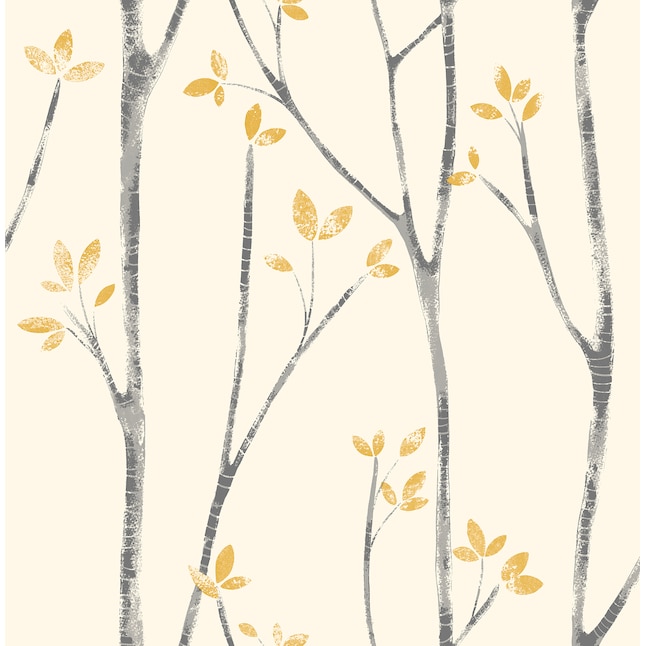The image depicts an artistic rendering of sparse shrub branches which extend vertically and horizontally across the canvas, even stretching beyond its borders. The branches, depicted in a darker shade of brown with lighter brown highlights, carry leaves at their tips. These leaves appear in a comparatively lighter brown shade, almost blending with the beige background that serves as the lightest color tone in the entire image. The composition suggests a minimalist, wallpaper-like pattern that features vertical lines of slender tree branches with subtle golden-brown leaves, positioned in various orientations – some reaching north to south and others south to north. The overall aesthetic presents a serene, nature-inspired design suitable for accent walls, emphasizing the delicate interplay between the branches and their softly highlighted leaves.